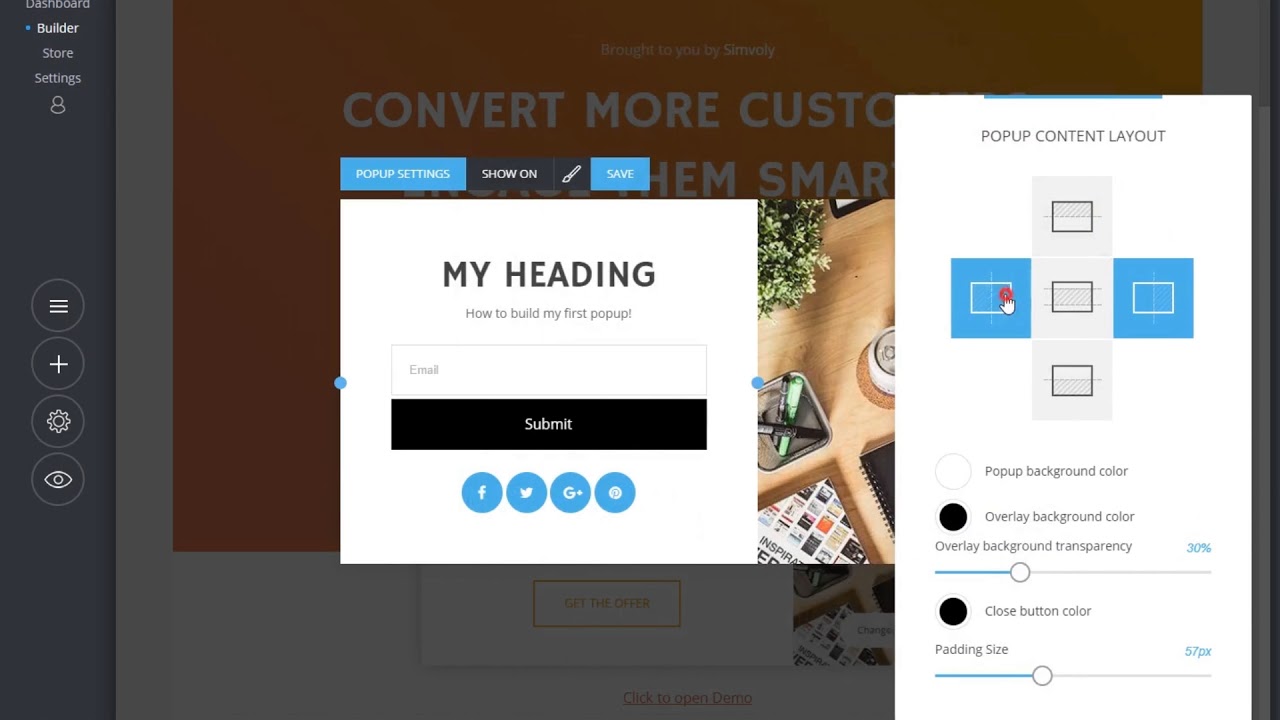The image depicts an interface of an e-commerce website builder. The left side of the screen features a dark gray sidebar with white text, listing options such as "Dashboard," "Builder," "Store," and "Settings." At the top of the sidebar, there's an icon resembling a person, likely representing the user account.

In the center of the webpage, a white pop-up window commands attention. This window is titled "My Heading" in black text. Directly beneath this heading, it reads "How to Build My First Pop-Up," suggesting that the user is in the process of designing a pop-up for their website. The central part of the pop-up includes a text entry field labeled "Email," accompanied by a "Submit" button below it.

To the right of the pop-up, a tall white box is visible, titled "Pop-Up Content Layout." This section appears to guide the user through arranging the content of their pop-up. The image reflects a user-friendly, interactive interface designed to facilitate the creation and customization of e-commerce websites.